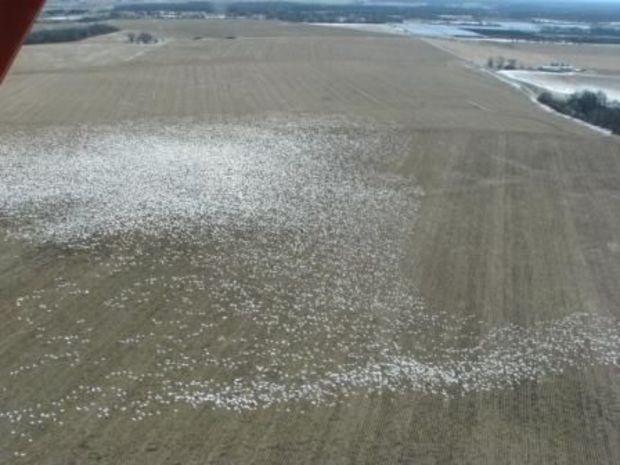This aerial photograph, possibly taken from a drone, airplane, or helicopter, showcases an expansive field with a mixture of green grass and brownish-gray soil, interspersed with irregular clusters of white patches. These patches are spread unevenly, with the largest concentration on the left side of the image, and additional rows of clumps extending towards the bottom right. The landscape appears worked, evidenced by visible rows and texture variations in the field. Up towards the horizon, particularly in the upper right corner, there are clusters of trees and a small pond, with a body of water – perhaps an ocean with a beach and white waves – visible further in the distance. The presence of a black diagonal bar and what may be a red component in the upper left suggest parts of the aircraft or drone that captured this image, adding to the context of a bird's-eye perspective. The photograph is detailed with various land features, foliage changes, and distant water bodies, creating a rich, layered landscape composition.